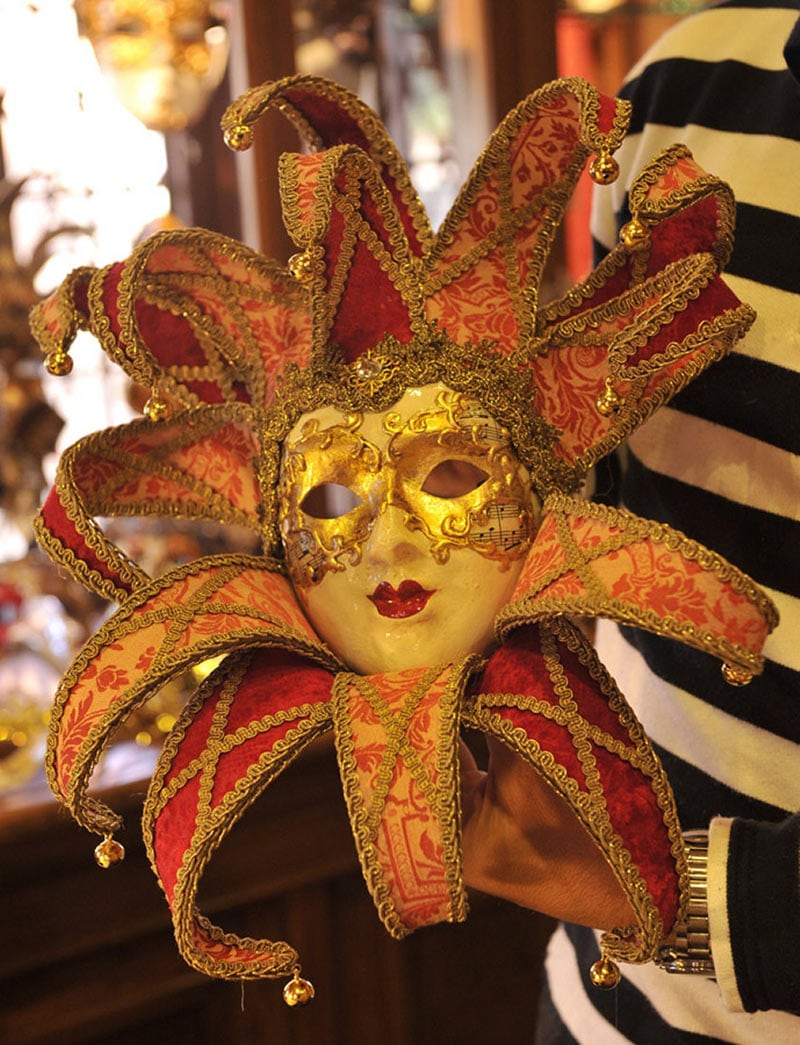The image features an elegantly designed mask that exudes an air of sophistication and theatrical flair. The mask is primarily gold, giving it a shiny and opulent appearance, accentuated by intricate red pendants on the sides and ornate gold accents throughout. The eyes are meticulously cut out, suggesting that this mask was intended for a specific wearer, possibly a physician. The base color of the mask is a mix of whitish-yellow, adding to its antique, circus-like charm, reminiscent of an old-style joker.

The lips of the mask are deeply puckered and vividly red, adding a striking contrast to the gold and whitish-yellow tones. A person holding the mask is visible, distinguished by their black and white striped shirt and a notable silver watch on their wrist. In the background, several other masks can be seen, enriching the scene with a sense of mystery and grandeur.